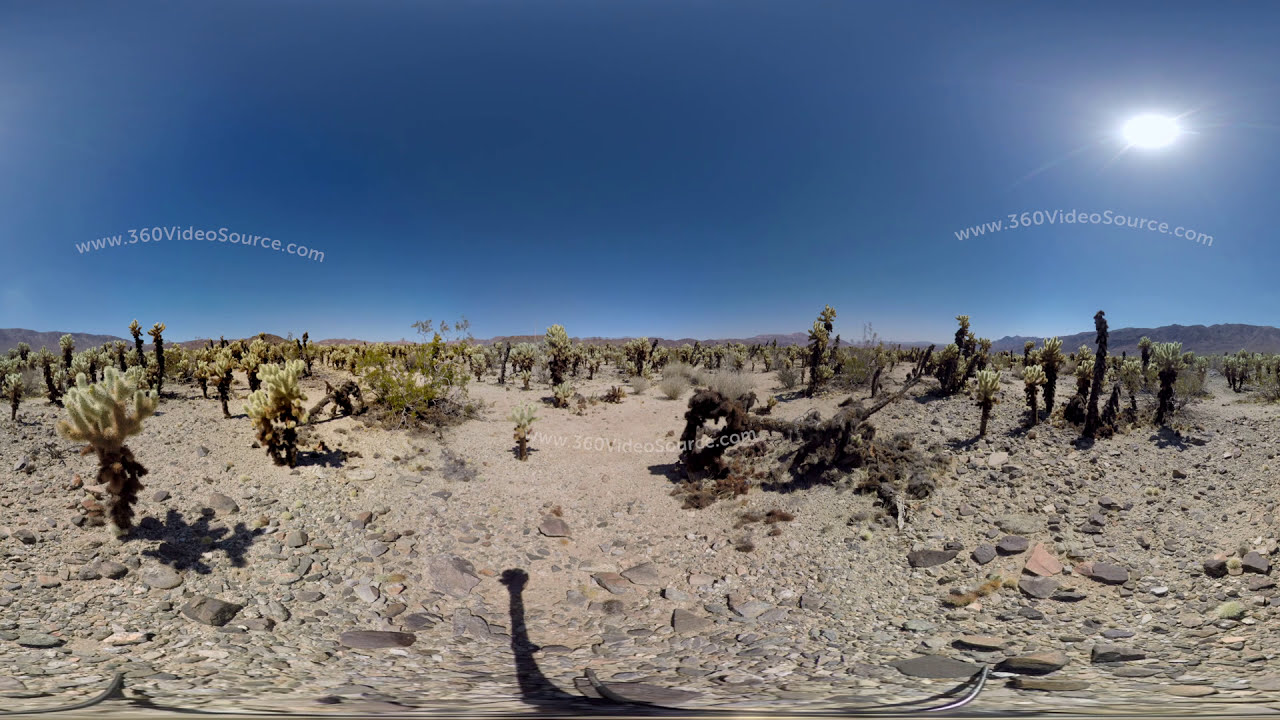The image depicts a vast desert landscape in a wide, horizontal rectangle. The top half showcases a bright blue sky with the glowing sun positioned just below the upper right-hand corner. The lower half reveals a barren expanse of grayish tan sand, interspersed with dark gray and brown rocks. Green cactuses, dotted with tiny thorns, rise from the ground, some reaching about the height of a person, alongside sporadic brush. In the distance, dark gray mountain ranges outline the horizon. A prominent log, brown and black in color with some plants growing on it, sits in the middle of the scene. The image has overlays of the text "www.360videosource.com" in white letters, with two instances across the sky and one across the sand and log. A subtle shadow of a hand, likely from the person taking the picture, is visible, emphasizing the outdoor, desert environment.